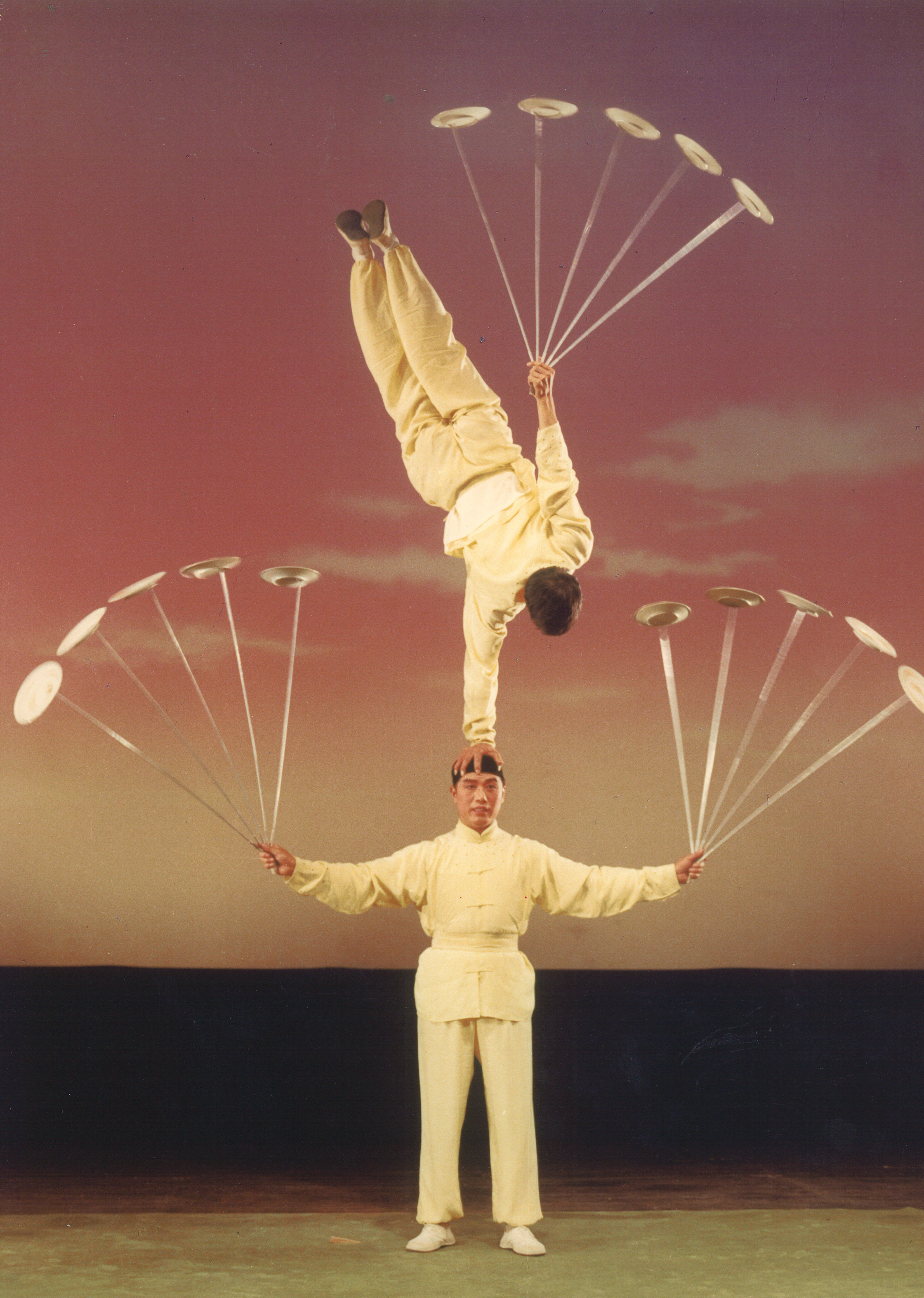This detailed vertically rectangular image captures a stunning acrobatic performance by two Chinese acrobats, dressed in coordinated white costumes with tight belts, white jerseys, and matching pants and shoes. The scene takes place indoors on a white stage, framed by a vibrant pink and white background with a dark border at the bottom.

The focal point of the image features one acrobat standing firmly on the stage, directly facing the camera, his arms extended outward. In each hand, he skillfully balances four sticks, each with plates twirling on top. Above him, the second acrobat performs an incredible feat of balance and strength, using only his right hand atop the standing acrobat's head to support himself. His body is stretched upwards, with his legs pointed slightly to the left and his head upside down. Like his partner, he too holds four similar plate-topped sticks in his free left hand. The performance, captured in full color and detail, highlights the precision, grace, and coordination of these skilled entertainers.